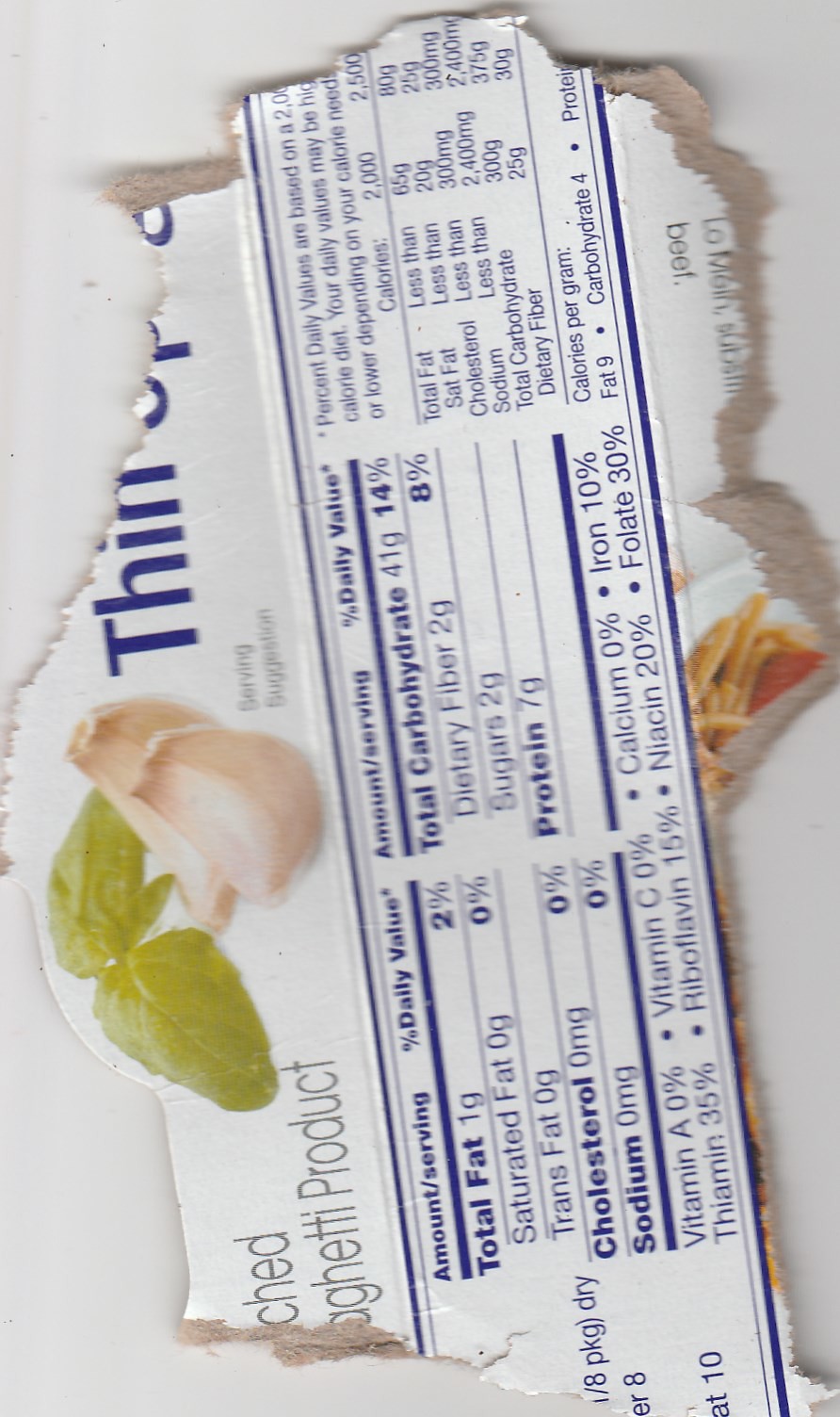A close-up, color image set against a light gray background in portrait orientation showcases a torn piece of cardboard packaging with ragged edges displayed vertically. On the upper left corner of the packaging, partial lettering reads "C-H-E-D" with some additional letters suggesting a type of spaghetti product, potentially "A-G-H-T-T-I." Central to the label are two leaves and an illustration resembling nuts, indicating perhaps an enriched or bleached variety. To the right, the fragmented word "thin" is visible alongside a portion of what seems to be the start of "S-P" and another letter. Detailed nutritional information is presented on a white background with blue text, listing one gram of total fat, zero grams of saturated fat, and 0% daily values for Vitamin C and Vitamin A, among other details.